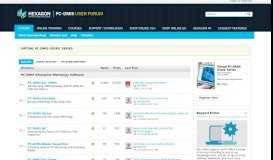The image showcases a highly zoomed-out section of a website's interface. The top portion of the site features a black background, with a search bar positioned on the right-hand side. On the left, the name of the website is displayed prominently. Beneath the website’s name, there are nine categories listed in small white text, with the first category highlighted in light blue. A light blue rectangle spans horizontally under these categories, delineating them from the rest of the page. Below this section, there are lines of small black text and an array of different categories. On the left side, there are sentences accompanied by numerical data arranged in rows, followed by additional links. To the right of these elements lies a small light gray rectangle with a blue settings icon. Beyond this, a vertical black bar stretches from top to bottom. The background of the lower half of the image is white, contrasting with the other elements present.